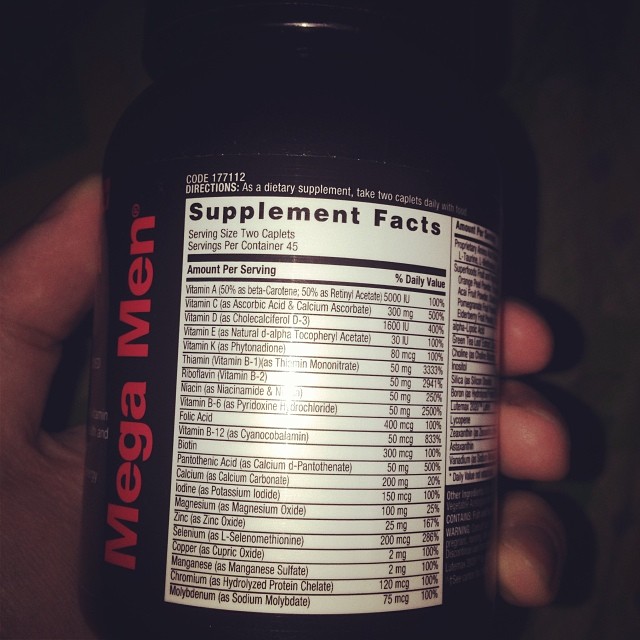The photograph showcases a dark-colored bottle of Mega Men supplements being held in a man's left hand. The backdrop is equally dark, making the illuminated label the focal point thanks to the camera flash. The name "Mega Men" is prominently displayed in large red letters running vertically along the left side of the bottle. The visible section of the label is the supplement facts, listing a serving size of two caplets, with 45 servings per container. Detailed information on the vitamins and minerals included in the supplement is provided, featuring Vitamin A, C, D, E, K, several B vitamins, calcium, iodine, magnesium, zinc, selenium, copper, manganese, chromium, molybdenum, and folic acid. The man’s hand, particularly the tips of three fingers, can be seen gripping the bottle.